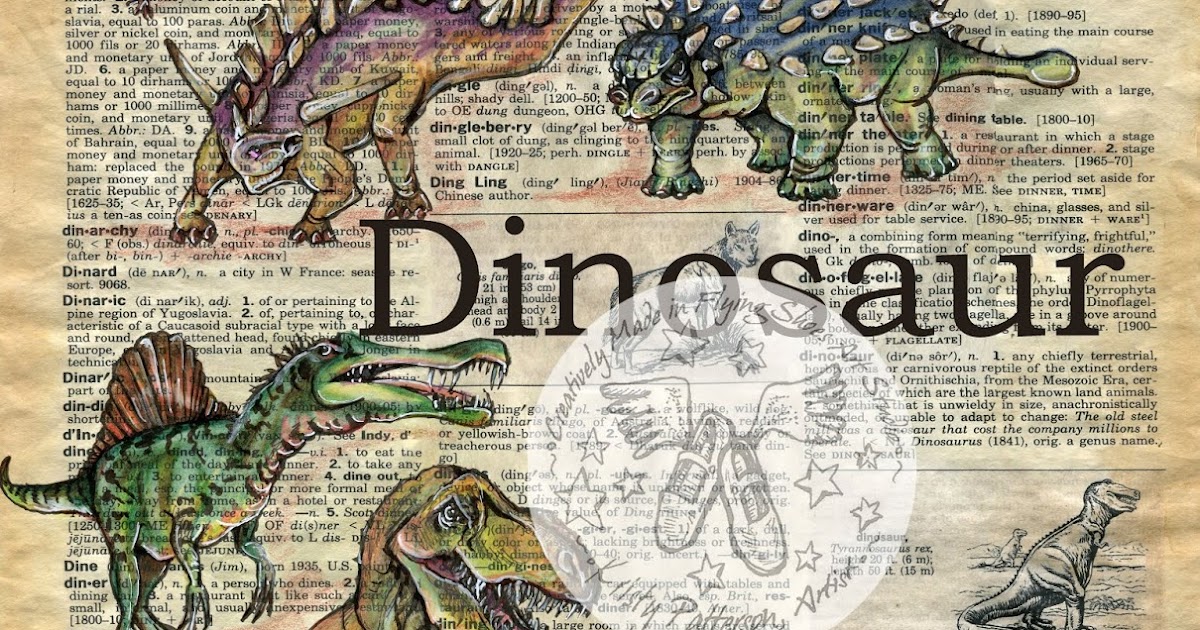The photographic image intricately layers several elements, centering on an old, yellowed dictionary or newspaper page that is slightly crumpled and worn, adding a vintage feel. The background consists of three columns of text with visible words and definitions, including "dinol," "dinoflage," "Dinaric," "dingo," "dingleberry," and various descriptions of monetary units and anthropological terms. Overlaying the text are vibrant, colorful illustrations of dinosaurs, each depicted with specific details: a green Ankylosaurus with a tail knob and numerous spikes, a Stegosaurus with a small head and distinctive spikes, a peculiar tyrannosaur-like dinosaur with a beak and fins, another resembling the head of a Tyrannosaurus rex, and a black-and-white depiction possibly of the same. At the top of the page, the word "Dinosaur" is prominently displayed in bold black font, emphasizing the theme. Adding an artistic touch, an inlaid graphic featuring a pair of winged shoes and the phrase "Creatively made in flying shoes by our Sinfonia, our strange Christy Patterson artist" is superimposed amidst the dinosaurs. This intricate amalgamation of vintage text and vibrant, animated dinosaur illustrations creates a detailed, compelling visual narrative.